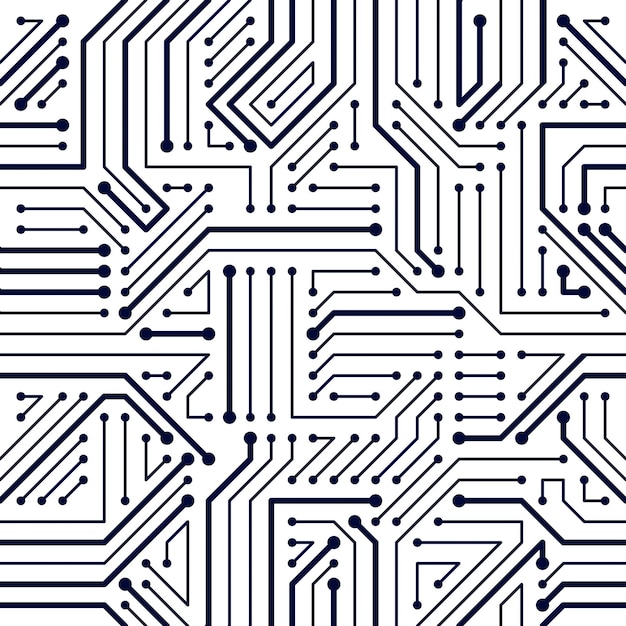The image depicts a complex, black-and-white, geometric pattern reminiscent of computer motherboard connections. Against a white background, an array of deep navy blue or black lines of varying lengths and widths extends in all directions—vertical, horizontal, angled, and bent. At the end of each line is a small, filled-in circle, though some lines around the edges are simply flat, ending at the frame. The design is highly symmetrical and maze-like, and appears both elaborate and ordered, evoking the intricate pathways found in electronic circuit layouts. The lines vary in thickness, with some connected and others isolated, suggesting a sophisticated, technical illustration that could serve as a pattern for wallpaper or another design purpose.